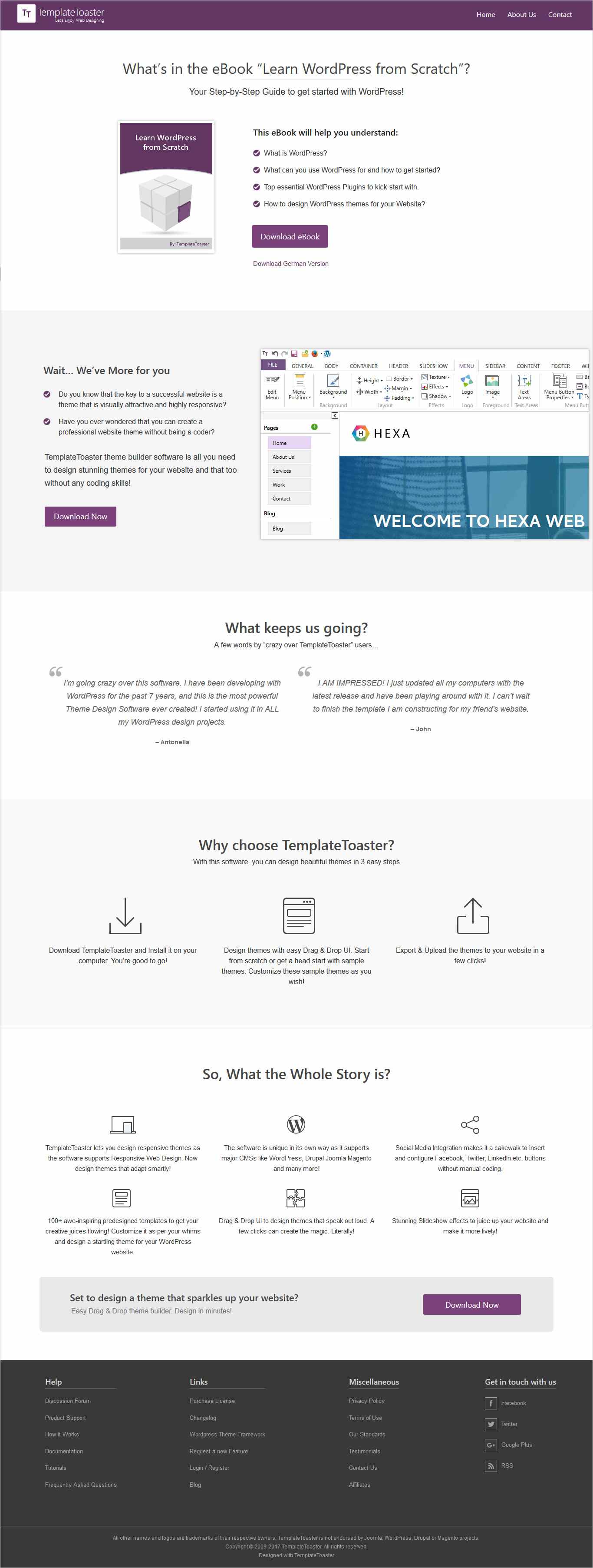This screenshot captures a webpage, likely an "About" or product description page for a website. The page has a clean, white background. 

At the very top, a purple banner stretches across the page, featuring a small logo positioned at the top-left corner.

Centered on the white background, there's a prominent heading that reads "What's in the Ebook: Learn WordPress from Scratch." Below this heading, on the left side, there's a thumbnail image of the ebook. Adjacent to the thumbnail on the right, there are several bullet points outlining the ebook's contents.

At the bottom of this section, there's a purple button for purchasing the ebook.

Beneath this section, a very light purple box contains descriptions of another product, accompanied by another purple button to purchase it.

Further down the page, a section titled "This is What Keeps Us Going" showcases customer quotes from reviews.

Following the customer quotes, there's another section titled "Why Choose Template?" This part includes three icons, each with a corresponding statement beneath them.

At the very bottom of the page, a section titled "So What the Whole Story Is" presents six different icons, each with descriptions below.